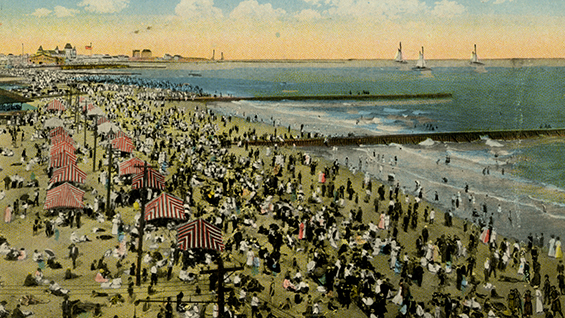The image is a detailed painting of a bustling 1920s beach scene viewed from a high vantage point. The beach, covered with people dressed in period attire—predominantly white, with large hats—is crowded with both beachgoers and swimmers in the water. Two long piers extend from the foreground out into the ocean. The sand is dotted with red and white striped tents set up in rows, as well as several umbrellas. In the background, three sailboats are visible gliding across the water, and further to the left is a harbor with structures that hint at a possible amusement area. Overhead, electric poles stretch across the scene, and the sky transitions from a golden hue near the horizon to light blue with fluffy white clouds at the top. Waves crash gently against the shoreline, completing this vivid and lively seaside depiction.